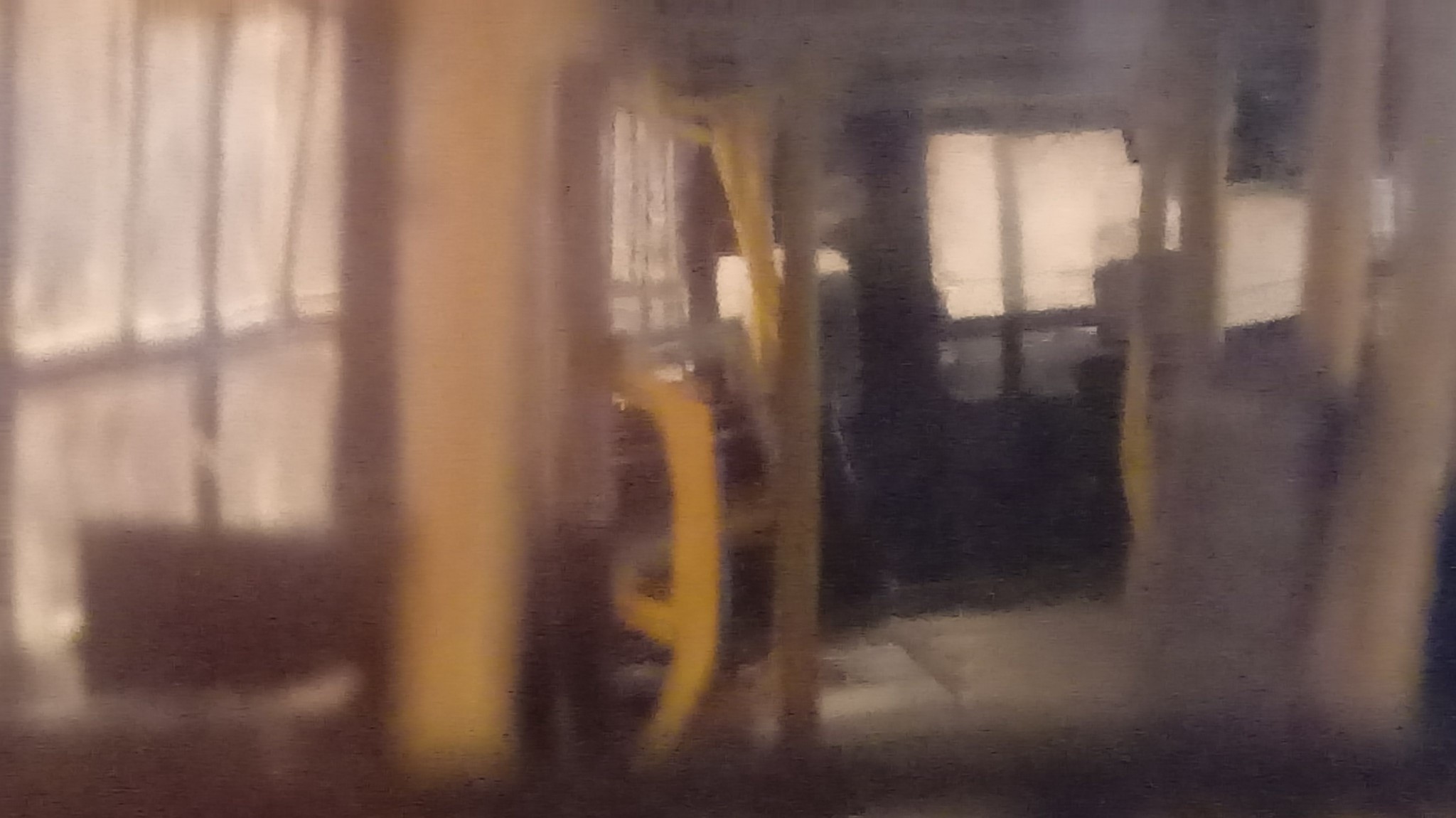The image captures a blurry, possibly interior scene, that seems to be undergoing construction or remodeling. The space is framed by beige and tan pillars on both sides, with a distinguishable curved yellow handle attached to one central pillar. The left side of the image features a line of windows that emit white light, shining through unwashed and dirty glass. In front of these windows stands a yellow pillar, accompanied by what appears to be a black and dark gray seat. The floor beneath is grayish in color. On the right side, additional beige pillars are visible, along with a dark gray object. The entire scene is suffused with a white haze, complicating the identification of details, but giving the impression of a room with construction-support structures resembling poles or beams reaching from floor to ceiling. Further into the room, there are more windows that suggest a larger, open space.